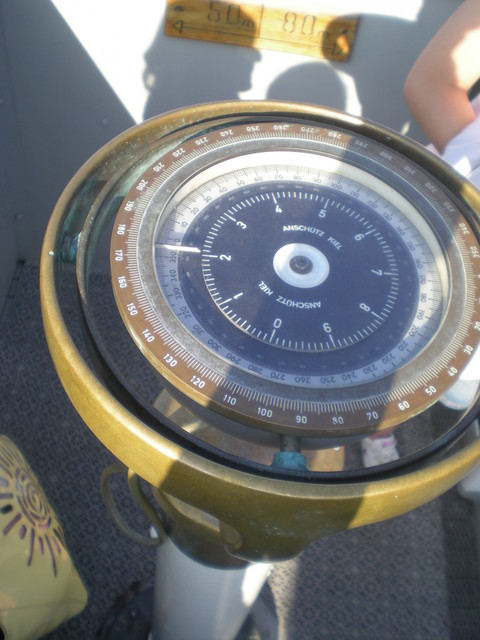This photograph appears to be taken outdoors, evident from the presence of shadows cast by the sunlight. The focal point of the image is a prominently displayed, round object occupying the majority of the frame. At the center of this object are the words "Ann Schuetz Kiel," though the pronunciation of "Kiel" is uncertain. The outermost portion of the object has a metallic, bronze-like appearance, and it encircles several layered, concentric rings.

One of these bronze rings is marked with numerical increments, starting at an indeterminate point but clearly readable from 30 through 310, increasing by tens. Between these numbers, small hash marks are present for finer measurement. Within these concentric circles are various gauges. 

Prominently in the center lies a round, white area adorned with further numerical markings. This central section features a substantial blue circle, embellished with the numbers 0 through 9, surrounding the "Ann Schuetz Kiel" inscription. 

In the background, a white wall is visible, adorned with a plaque or similar fixture. The presence of people nearby is suggested by the shadows of heads cast against the white wall, hinting at human activity surrounding the scene.